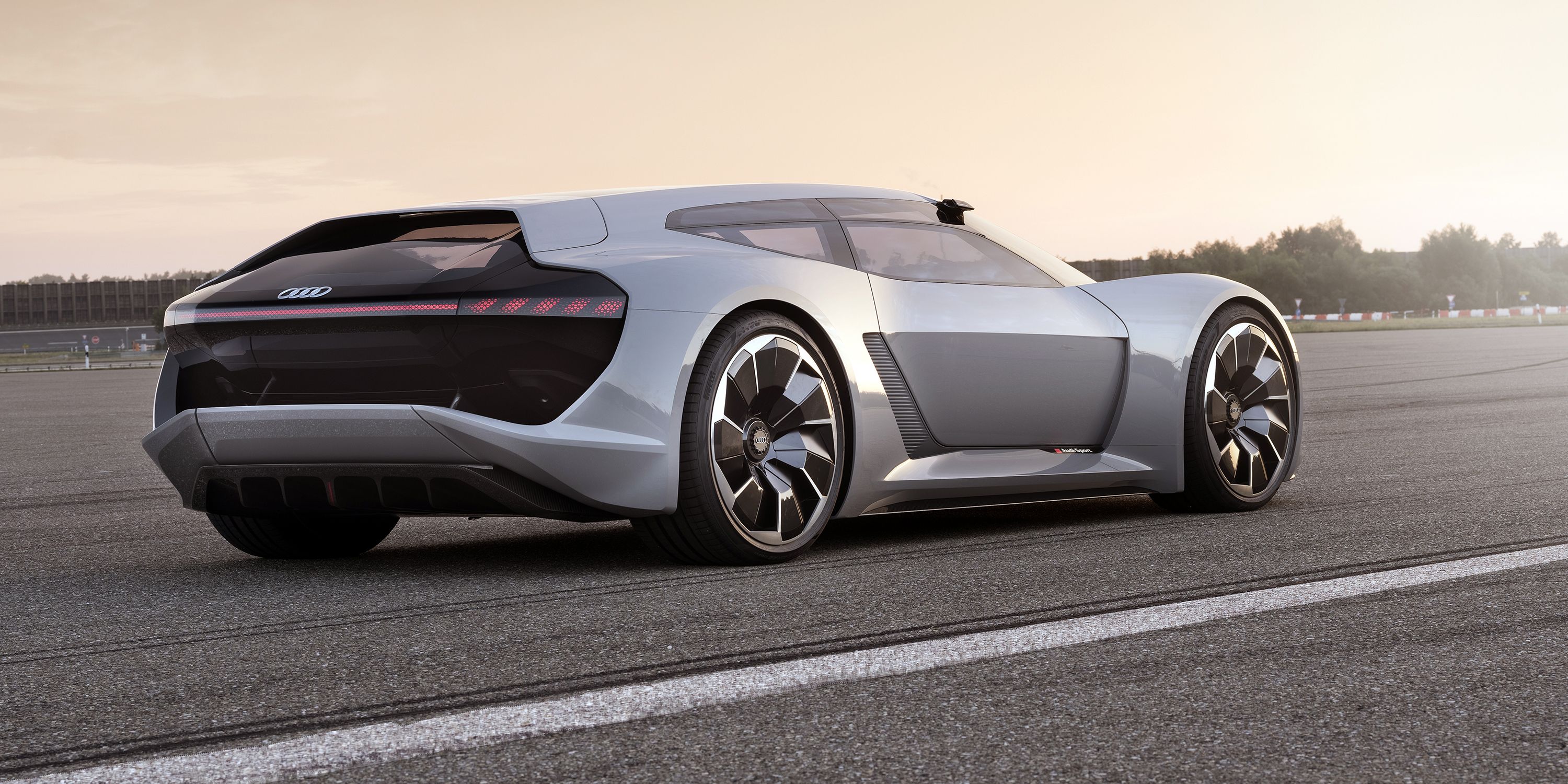This vibrant, horizontally oriented photograph captures a sleek, silver Audi sports car from the rear right angle, parked on a blackish-gray pavement—possibly finely packed dirt or concrete—on what appears to be a racetrack or stadium setting. The car is striking with its low-slung, aerodynamic design, featuring black and silver chrome wheels that fill the wheel wells entirely. The back of the car transitions from silver to black, adorned with the distinctive four-ring Audi logo and a set of red runner lights beneath. Above the car, the sky is cloudy but hints at sunrise or sunset, casting a low, ambient light over the scene.

A black, square object is noticeable on the right passenger window, adding to the car's sophisticated look. In the background, a white and red fence stretches out, likely marking the perimeter of the area, while a line of lush green trees adds a touch of nature to the otherwise industrial locale. Several buildings are also visible, enhancing the sense of a professional testing ground or a photo shoot setting. A thin white line on the pavement in front of the car and racing flags in the distance hint at a sport or track environment, suggesting the car is poised for either a promotional shoot or a high-speed test drive.